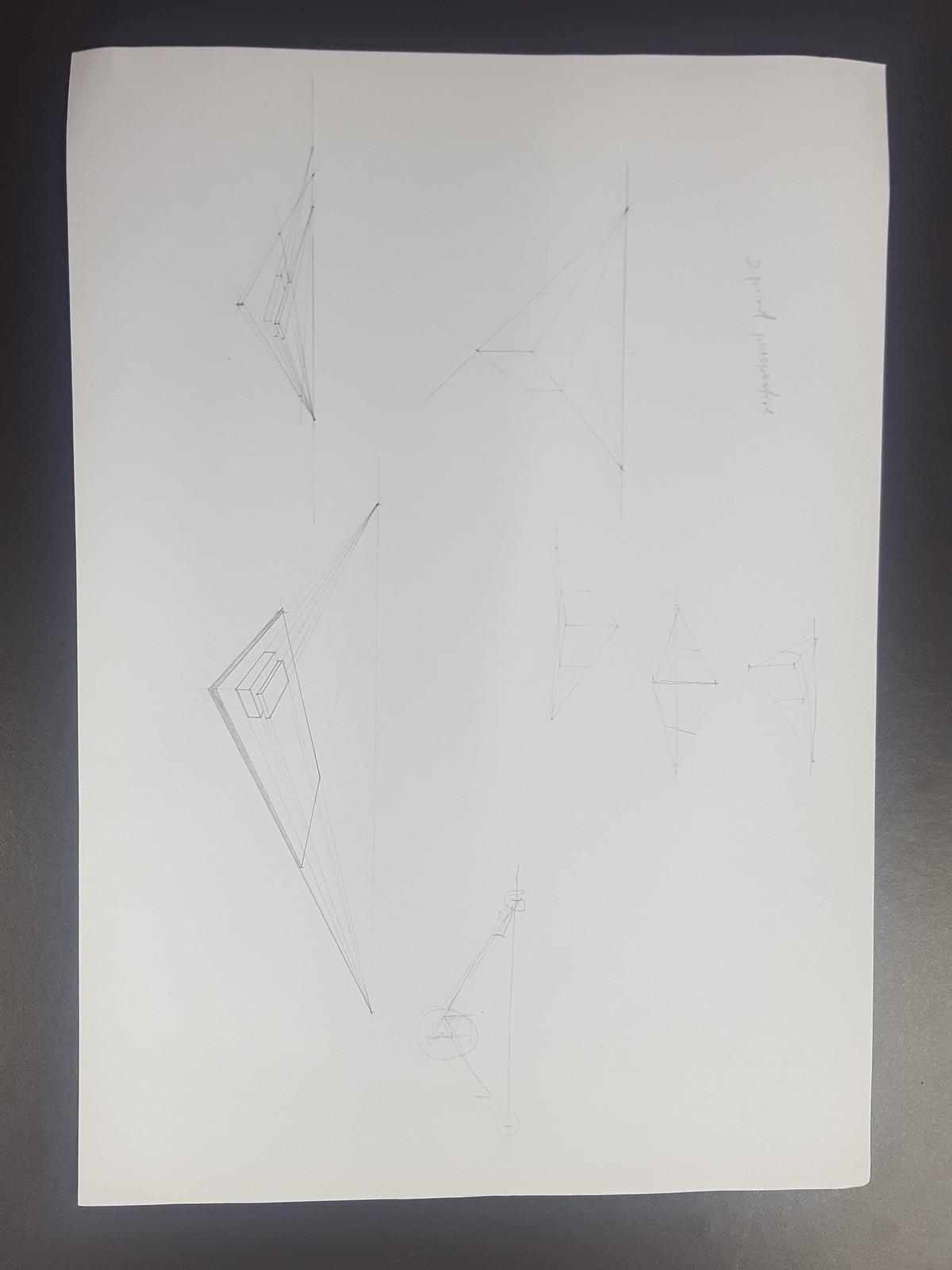This image features a pencil drawing on a sheet of white paper, positioned sideways on a black platform. The drawing is indistinct due to the low quality of the image, making it difficult to discern specific details. The artwork seems faded, adding to the challenge of interpretation. In the top right corner of the paper, there is some writing, but it is too blurry to read. To the left of the sheet, there is a clearly visible drawing of a triangle. The overall lack of clarity in the image impedes further detailed identification of the drawing.